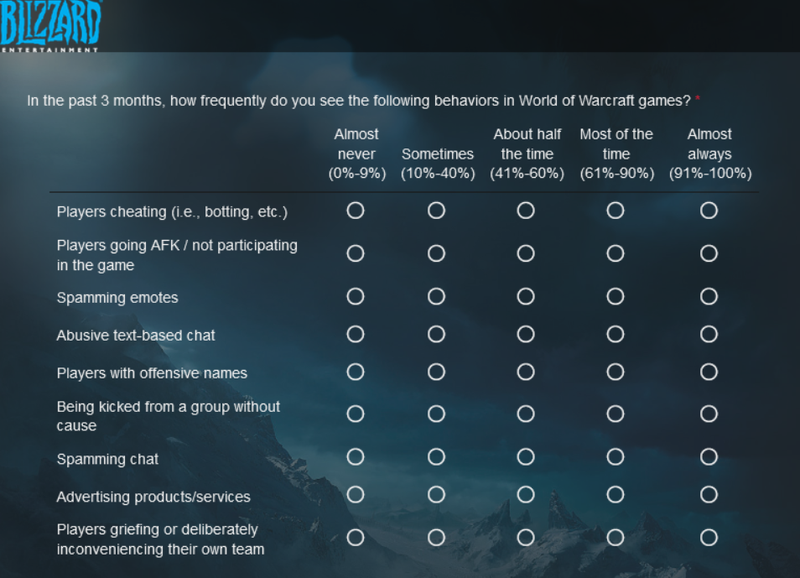The image is a detailed landscape illustration that doubles as a survey form related to players' experiences in World of Warcraft. In the upper left-hand corner, the light blue logo of Blizzard Entertainment is prominently displayed. This logo is isolated in a top stripe with no other content.

The background of the form features a deserted planetary landscape with noticeable elements: sparse clouds, numerous rocks, and towering mountains, adding to the desolate ambiance. 

At the top of the form, bold white text poses the question: "In the past three months, how frequently do you see the following behaviors in World of Warcraft's games?" Below it, the survey offers choices for respondents to select based on their experiences: almost never, sometimes, about half the time, most of the time, and almost always. 

The left side of the form lists various in-game behaviors that players may encounter:
- Players cheating
- Players going AFK (away from keyboard) and not participating
- Spamming emotes
- Engaging in abusive text-based chat
- Using offensive names
- Being kicked from a group without just cause
- Spamming chat to advertise products and services
- Players griefing or deliberately inconveniencing their own team

Respondents are expected to choose the circle that aligns with the frequency they have observed each behavior.